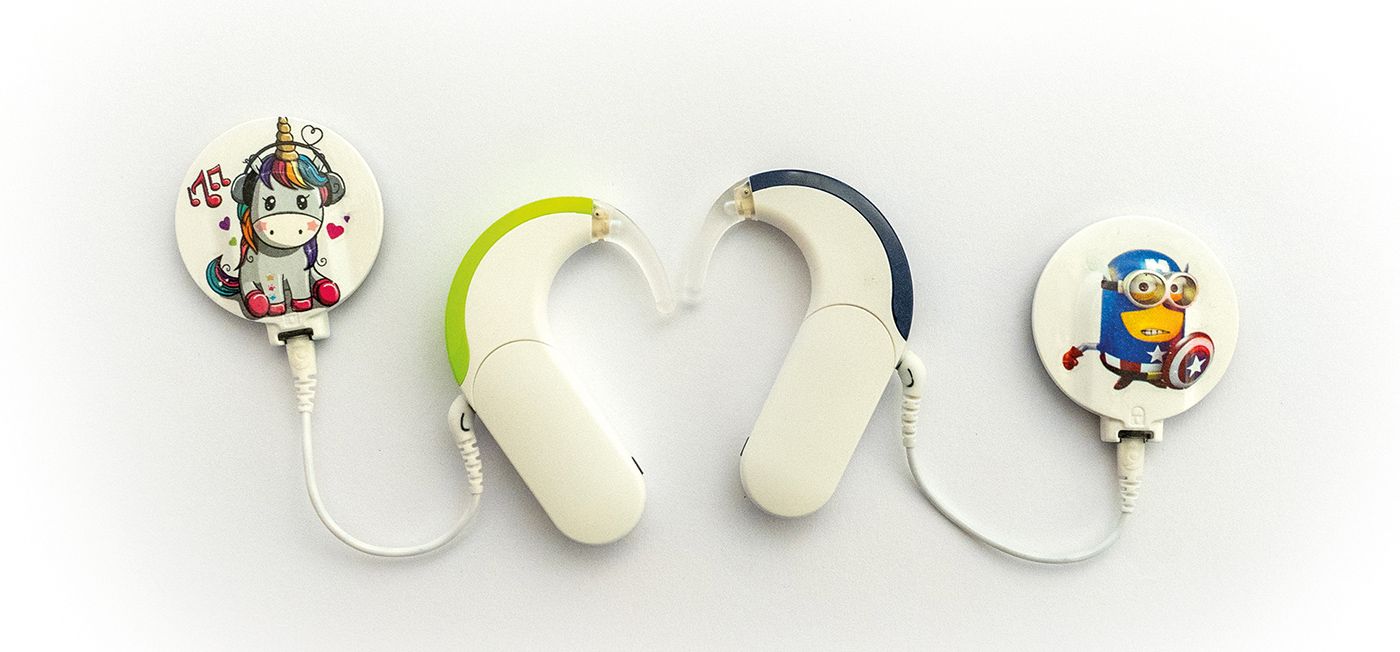The image features two children’s cochlear implants designed to resemble popular characters. The implants are positioned together to form a heart shape with their curved tops and bent bases. Each device has a wire trailing off to a circular magnetic base that attaches to the head. The implant on the left sports a neon green trim and features a colorful unicorn with a golden horn, rainbow hair, red feet, black headphones, and music notes. The implant on the right, trimmed in navy blue, showcases a Minion from "Despicable Me" dressed as Captain America, complete with a shield and goggles. Both implants are plugged in, forming a whimsical and functional accessory for kids.